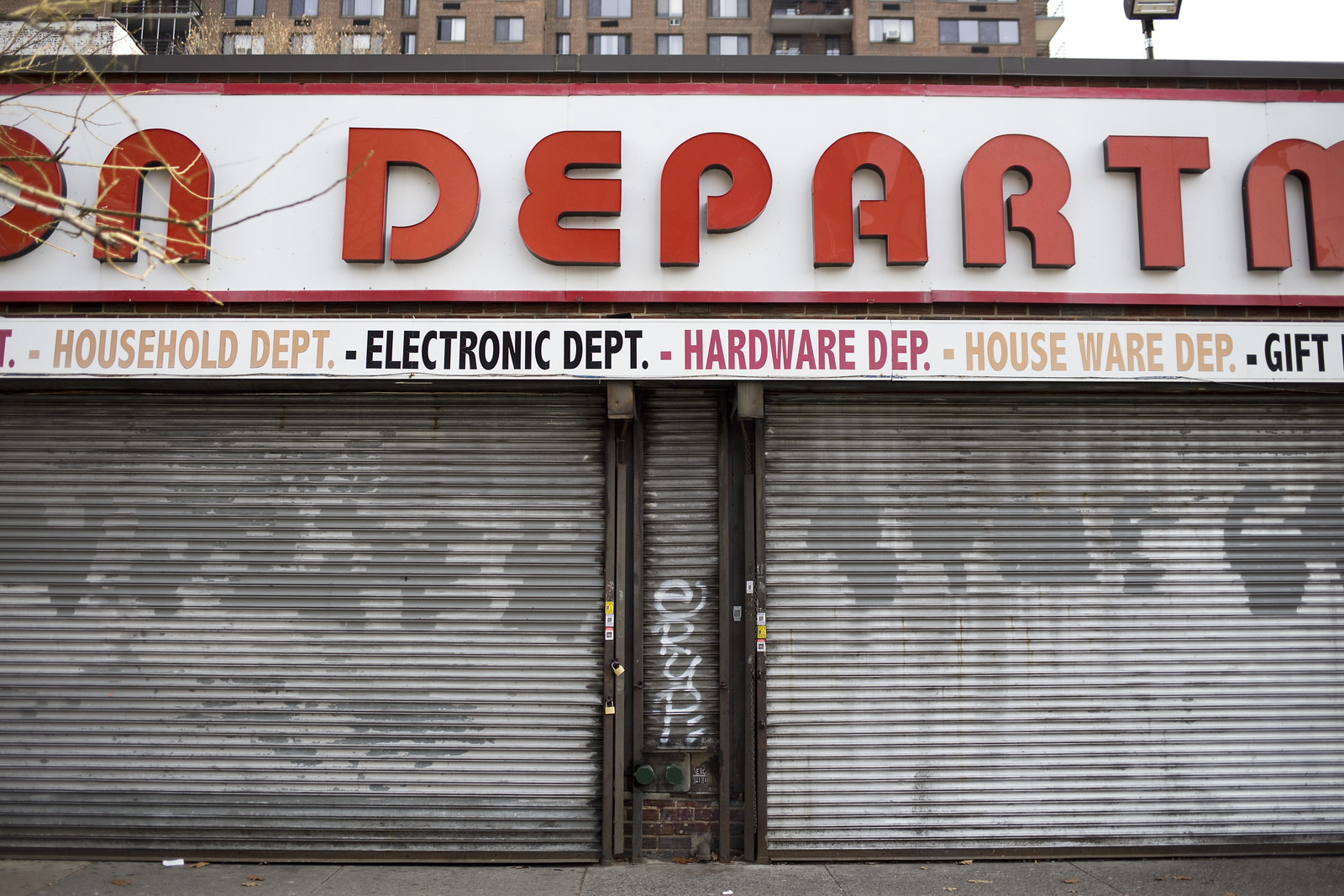This photograph depicts a storefront secured with metal, shutter-style gates, which have been pulled down to cover the windows. Gold-colored locks secure the entryways. The gates are silver, contrasting with the gray concrete ground in front of the store. Above the storefront is a partially visible white and red sign displaying the text "ONDEPARTM." Beneath this, another white sign lists the departments available: Household Dept., Electronic Dept., Hardware Dept., Houseware Dept., and Gift Dept. Each "Dept." is abbreviated as "D-E-P-T." The overall scene suggests the store is closed.